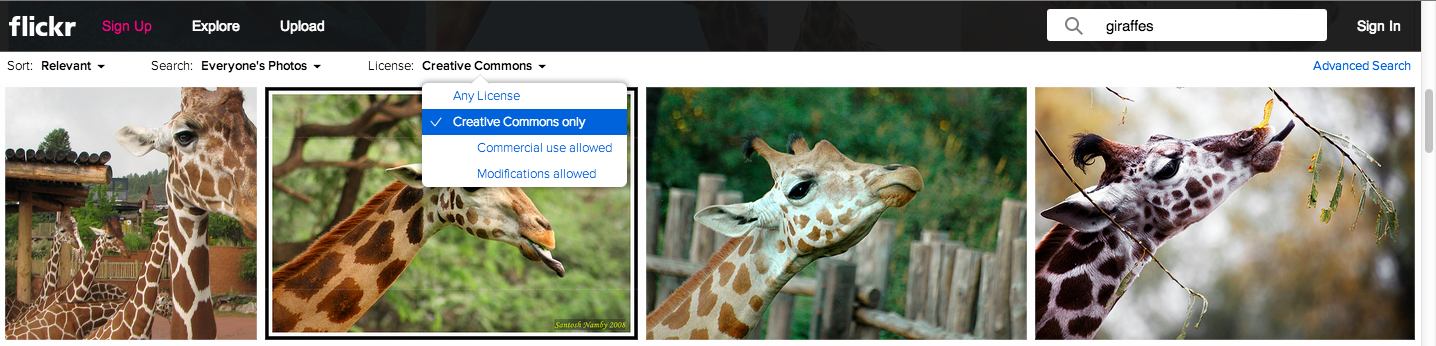In the image's top portion, it features a sleek black background with the word "FLICKR" prominently displayed in white, followed by "SIGN UP" in vivid pink. Adjacent to these are options labeled "EXPLORE," "UPLOAD," and "SORT VELVET" in white text. Below these, there is text prompting users to "SEARCH EVERYONE'S PHOTOS" and an option to "CREATE COMMENTS WITH LICENSE." A user has clicked on the "CREATIVE COMMONS" filter, which has turned blue with a white checkmark indicating selection. Under this filter, additional text reads "COMMERCIAL USE ALLOWED" and "MODIFICATIONS ALLOWED."

In the search box against the black background, the term "GIRAFFES" is entered, resulting in the display of four images of giraffes. The second image is partially obscured by a popup, but the other three are clearly visible. The first and third giraffes are simply standing still, while the fourth giraffe is captured with its tongue extended, seemingly trying to reach a leaf. The overall composition indicates a search on Flickr, showcasing both the interface elements and the resulting images related to giraffes.